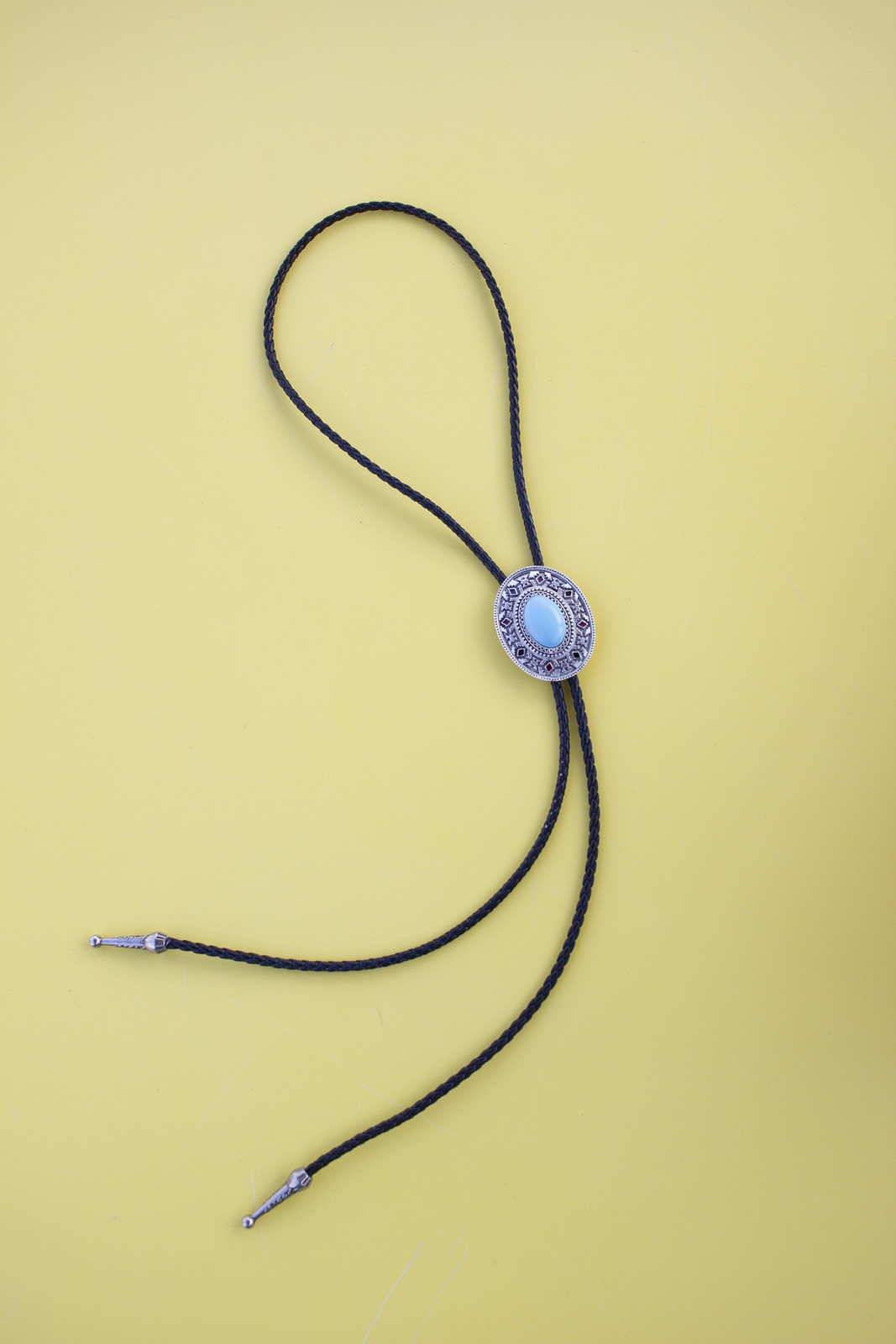This image showcases a Western-inspired bolo tie, meticulously photographed against a plain, pale yellow background. The bolo tie features a simple black braided cord, whose evenly spaced ends extend towards the bottom left corner, each tipped with thin silver pointed metal pieces. At the center of the cord, an ornate pendant acts as the tie’s centerpiece. This pendant is predominantly oval-shaped, with a light blue gem at its heart. Encircling the gem, a white plate embellished with dark blue geometric designs, including diamonds, triangles, and swirls, adds an intricate detail. The black cord loops through the pendant, enhancing the visual symmetry and balance of the piece.